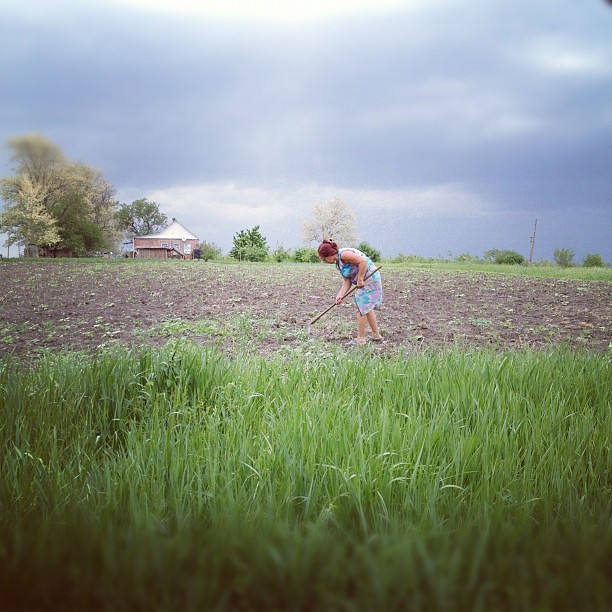The photograph depicts a woman with red hair, wearing a blue and purple floral-themed dress, working with a backhoe in an undeveloped field. The area closest to the camera is filled with overgrown grass, while the section where the woman is working comprises mostly bare earth with sparse vegetation. The woman, approximately 40 feet from the camera and facing left, is bent over, actively engaged in weeding or preparing the soil for planting. In the background, about 200 to 300 meters away, stands an old, small residential structure with both brown and white features, suggesting a rural setting. A power pole near the house further indicates the remoteness of the location. The sky overhead is overcast, filled with a mix of gray and white clouds, casting a somber tone over the scene.